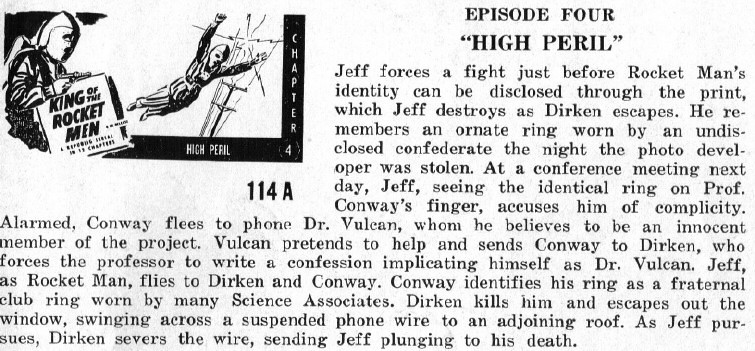The image is a scan of a book page, featuring a detailed layout with a body of text on the right and a small rectangular black-and-white cartoon on the left. The cartoon depicts two characters: one character appears to be jumping off the sail of a ship, while the character on the left holds a sign reading "King of the Rocket Men." Below this image is the identifier "114A." The text to the right bears the title "Episode 4 High Peril," with the phrase "High Peril" emphasized in a bolder font. The accompanying text reads: 
"Jeff forces a fight just before Rocket Man's identity can be disclosed through the print, which Jeff destroys as Durkin escapes. He remembers an ornate ring worn by an undisclosed Confederate the night the photo developer was stolen. At a conference meeting the next day, Jeff, seeing the identical ring on Professor Conway's finger, accuses him of complicity. Alarmed, Conway flees to phone Dr. Vulcan, whom he believes to be an innocent member of the project. Vulcan pretends to help and sends Conway to Durkin, who forces the professor to write a confession implicating himself as Dr. Vulcan. Jeff, as Rocket Man, flies to Durkin and Conway. Conway identifies his ring as a fraternal club ring worn by many science associates. Durkin kills him and escapes out the window, swinging across a suspended phone wire to an adjoining roof. As Jeff pursues, Durkin severs the wire, sending Jeff plunging to his death."